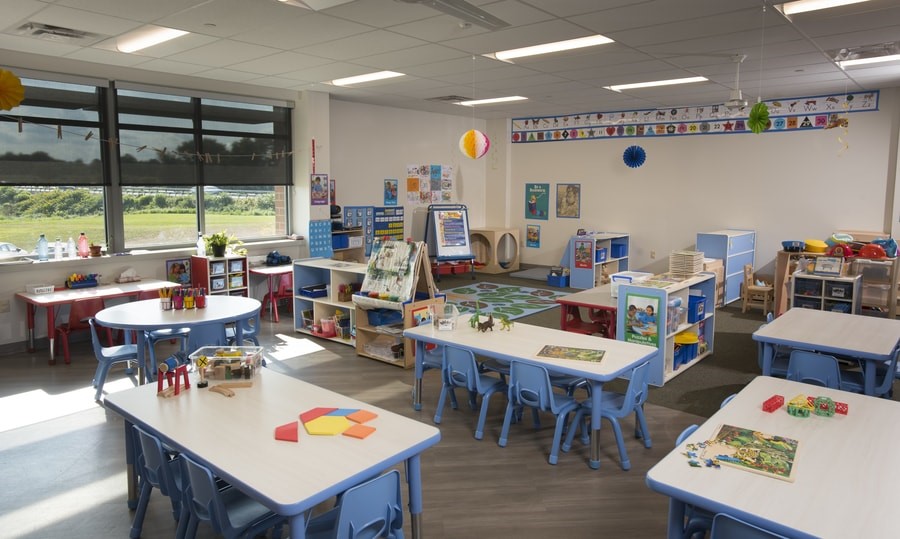The image captures a meticulously organized kindergarten or daycare classroom, vibrant and designed to engage young children. The walls are adorned with educational posters, including an alphabet and numbers up to 30, contributing to the room’s learning-focused atmosphere. Colorful, balloon-like decorations hang from the ceiling, complementing the playful environment. The room features several white tables, both circular and rectangular, paired with baby blue plastic chairs. Different stations are set up throughout the room, including a painting area with little cups of paintbrushes, a carpeted corner for activities like show-and-tell or read-alouds, and shelves filled with toys, puzzles, and art supplies. The bright, sunlit room benefits from natural light streaming through a large window with views of the sky and green grass outside, adding to the pleasant, cheerful ambiance. Despite the ample educational materials and creative work areas, the classroom is currently unoccupied, emphasizing its tidy and well-maintained state. Fluorescent lights in the ceiling ensure the space is well-lit, making it an inviting environment for young learners.